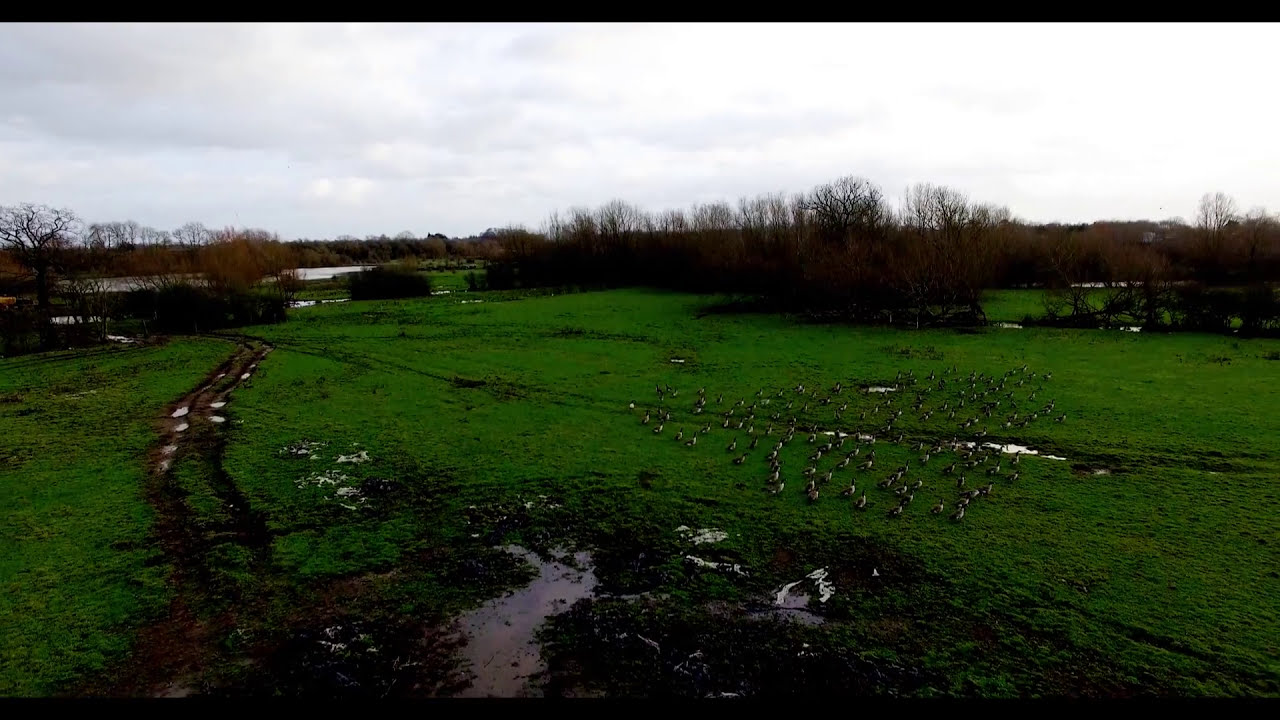The photograph captures a cloudy day in a countryside setting, dominated by a muddy field interspersed with green grass. Prominent muddy tire tracks traverse the landscape, leaving puddles of water and rivets in their wake, hinting at recent rainfall. Toward the right side of the field, a large flock of Canadian geese stands in the grass. In the background, leafless trees outline the horizon, suggesting a season of fall, winter, or early spring. The sky is overcast with white and gray clouds, casting a dim light over the scene. At the far left, behind the trees and bushes, there are faint outlines of structures or perhaps a shimmering body of water, adding depth to the composition. Long, thin black bars run horizontally across the top and bottom edges of the image, framing the serene but somber rural landscape.